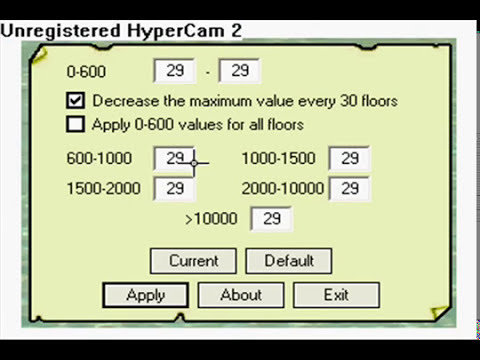The image is a screenshot of an unregistered HyperCam 2 software interface, possibly used for home valuation or by realtors. The main background color is green with a lighter green overlay that appears slightly folded at the top left and bottom right corners. There are simulated tears on the top and bottom edges of the overlay. At the top, it displays the range "0-600" with two number input boxes below it, both filled in with the number "29." Adjacent to these boxes is a checked checkbox labeled "Decrease the maximum value every 30 floors." Beneath that is an unchecked checkbox labeled "Apply 0-600 values for all floors." Further down, there are more range intervals: "600-1000," "1000-1500," "1500-2000," "2000-10000," and ">10000," all with "29" filled in the input boxes next to them. At the bottom of the screen, there are buttons labeled "Current," "Default," "Apply," "About," and "Exit." The interface uses yellow, white, and brown text, and the entire screen is framed by a black letterbox effect occupying about 5-10% of the image's perimeter.